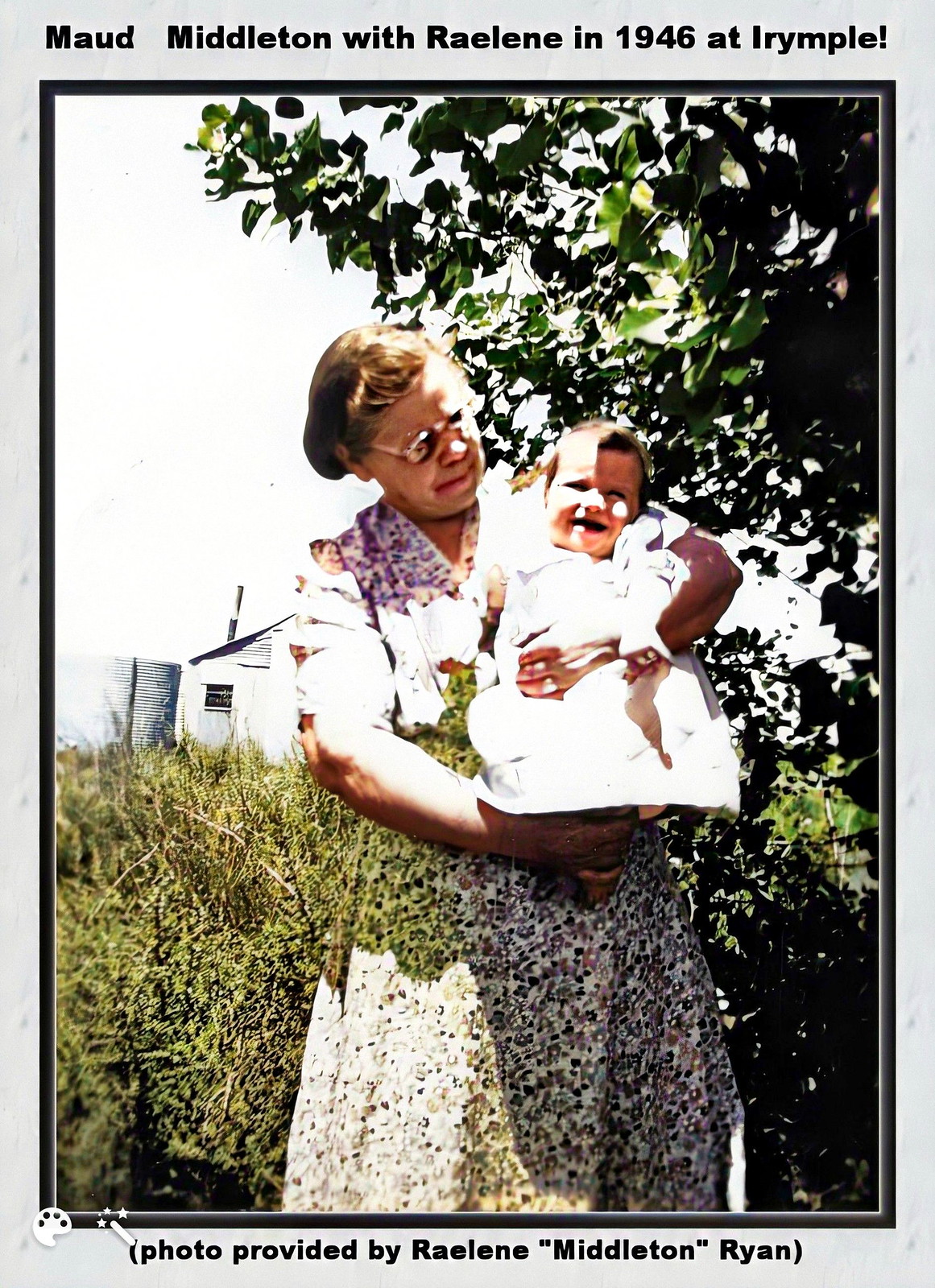The image is a vertically oriented card featuring a photograph bordered by a light gray frame, wider at the top and bottom than on the sides. The top border is inscribed with "Maude Middleton with Raylene in 1946 at Eye Ripple," while the bottom border reads "Photograph provided by Raylene Middleton 'Ryan'." 

The central focus of the photograph is a middle-aged to older woman, Maude Middleton, dressed in a flowery dress. She stands slightly right of center, facing forward with her head turned slightly to the right, gazing down at a baby. The baby, wrapped in a white blanket, also looks slightly to the right and appears to be smiling. Maude Middleton is holding the baby, identified as Raylene, who grows up to provide this photograph. 

In the background, you can observe a thick brush and a tree to the right. Far in the distance over Maude's right shoulder, there is a building and another structure to its left. The scene appears to be outdoors on a clear day, with the natural elements elegantly juxtaposing the subjects.